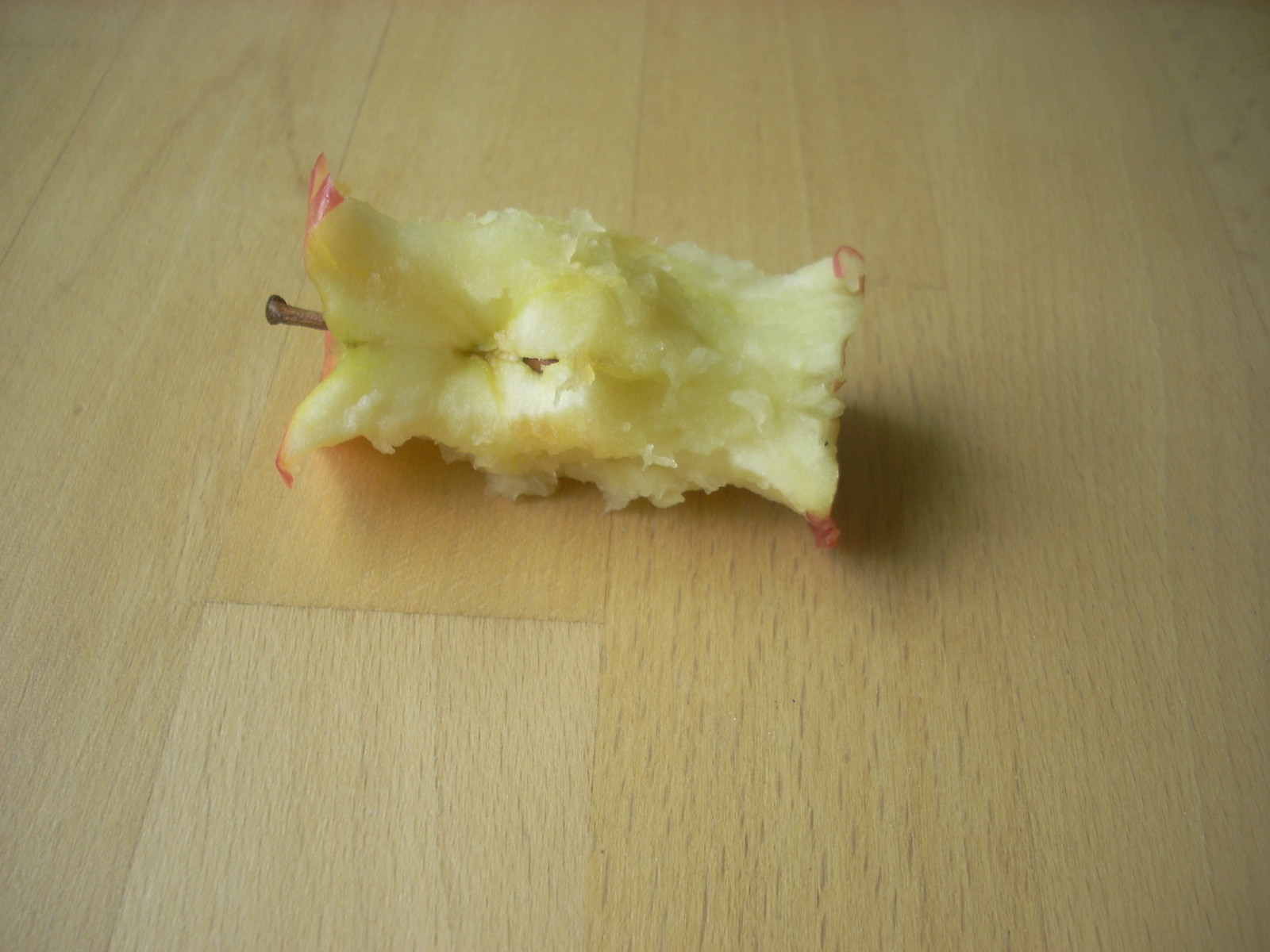A high-quality, zoomed-in photograph focuses on the partially-eaten core of a red apple. The remaining apple flesh, which is predominantly white with slight tinges of green, clings to the brownish core that extends horizontally across the image. At one end of the core, a small brown stem is visible. The remnants of the apple reveal thin, shiny, red skin at both the top and bottom, reflecting the light source in the scene. The apple core is situated on what appears to be a pale wooden or laminate floor, adding a naturalistic backdrop to the composition.